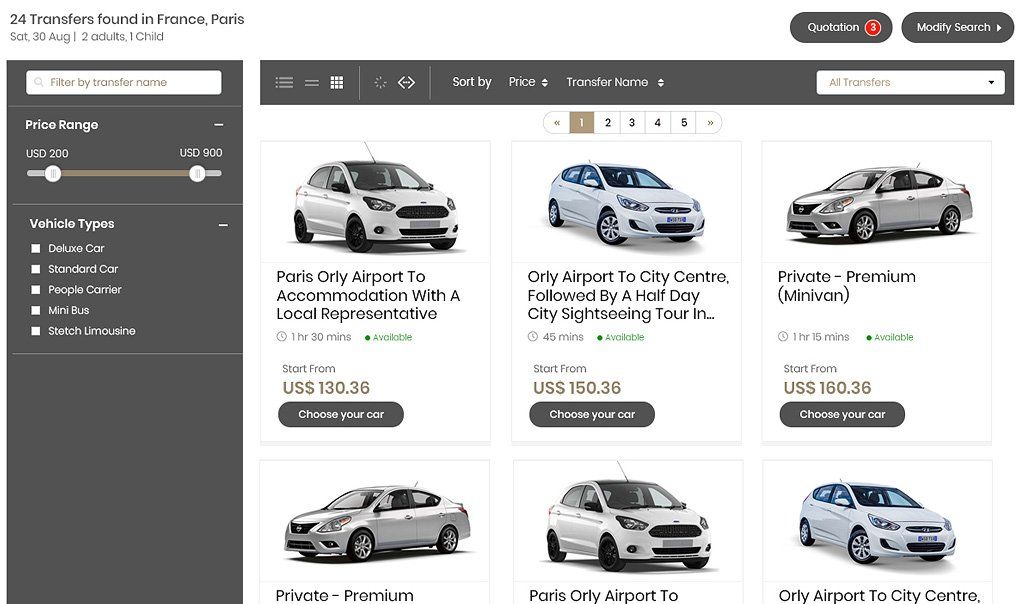**Caption:** 

"Explore convenient transfer options for your Paris trip: Available from Saturday, October to August, choose from a variety of vehicles including a deluxe car, standard car, people carrier, minibus, and stretch limousine. Transfers range in price from US$200 to US$900 and are listed by transfer name. For a seamless journey, options include general transfers as well as specific routes like from L.Y. Airport to Paris city center with a half-day private premium sightseeing tour. With rates starting at US$130.36, enjoy a 1 hour and 30-minute trip with a local representative. Thank you for watching and choosing your ideal transfer!"

---

This reformulation ensures clarity by organizing the details into a coherent and enticing description suitable for potential travelers looking for transfer services.